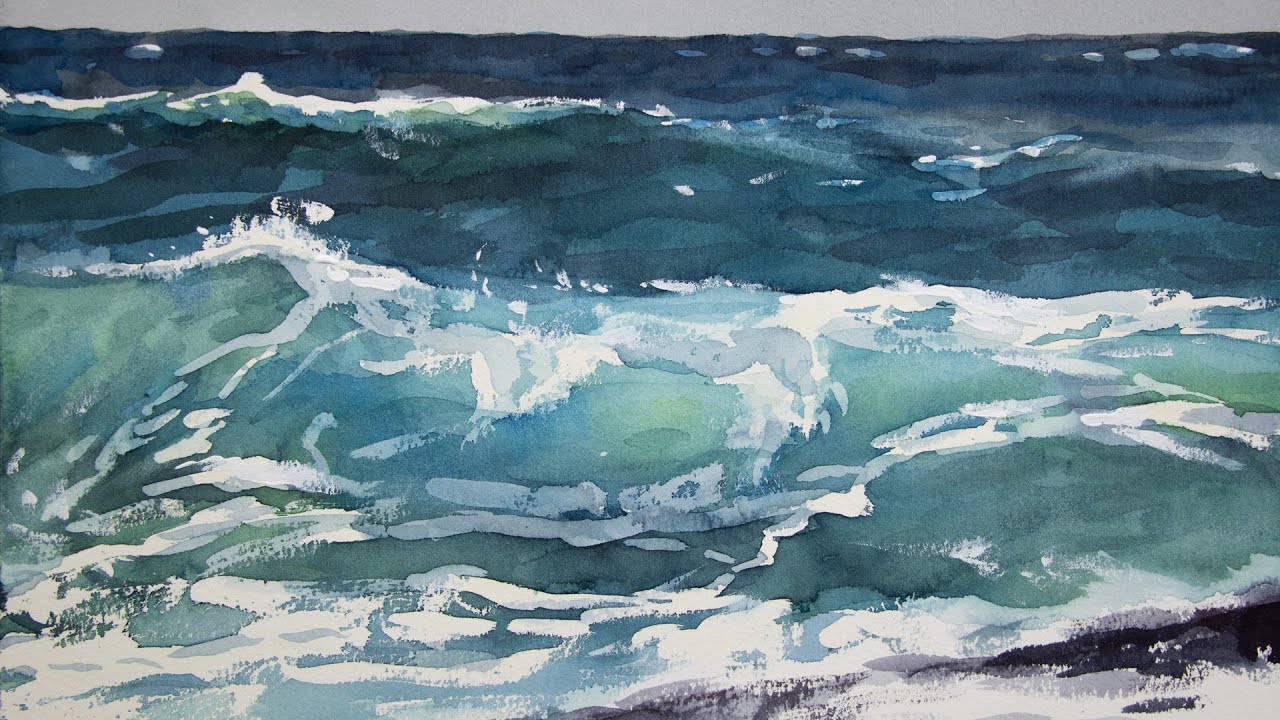This painting depicts a dynamic seascape with a narrow gray sky barely visible at the top. The ocean transitions from dark blue at the horizon to lighter blue and eventually a grayish-blue toward the front. Our viewpoint rests on the beach where waves roll in shallow and capped with white foam, poised to crash and spill onto the sand. The middle of the image features more turbulent, white-capped waves, highlighting the sea's varying depths and energy. The distant waves are darker, with patches of white foam, encapsulating the ocean's shifting hues and textures under the overcast sky.